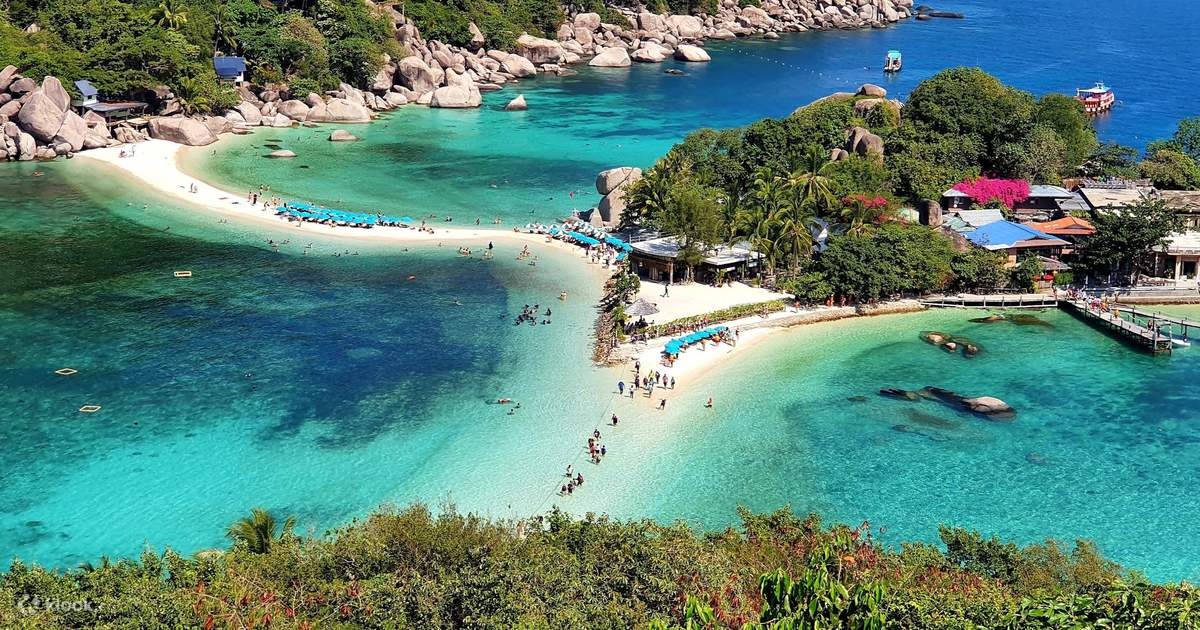This aerial view captures a stunning tropical landscape featuring three main islands interconnected by narrow strips of white sandy beach. The image is wider than it is tall, showcasing a picturesque beach in the foreground, dotted with vibrant turquoise lawn chairs and people engaging in various activities like walking, sunbathing, and swimming in the crystal-clear coastal waters. The water varies in color from bright turquoise near the shore to darker blues as it deepens.

To the right of the image, nestled among lush vegetation, is a small village or resort area with flat-roofed buildings and brightly colored rooftops. Several docks stretch out over the water, and a few boats are anchored nearby, enhancing the idyllic, vacation-like atmosphere. The middle island, slightly smaller but bustling with structures, features a prominent dock and numerous buildings. The backdrop includes a larger island covered in dense greenery and lined with rocks and boulders where the vibrant vegetation meets the radiant blue waters.

Overall, the photograph beautifully captures the harmonious blend of natural beauty and subtle human presence, from the verdant hill and rocky edges to the clear, inviting waters and lively beachfront.